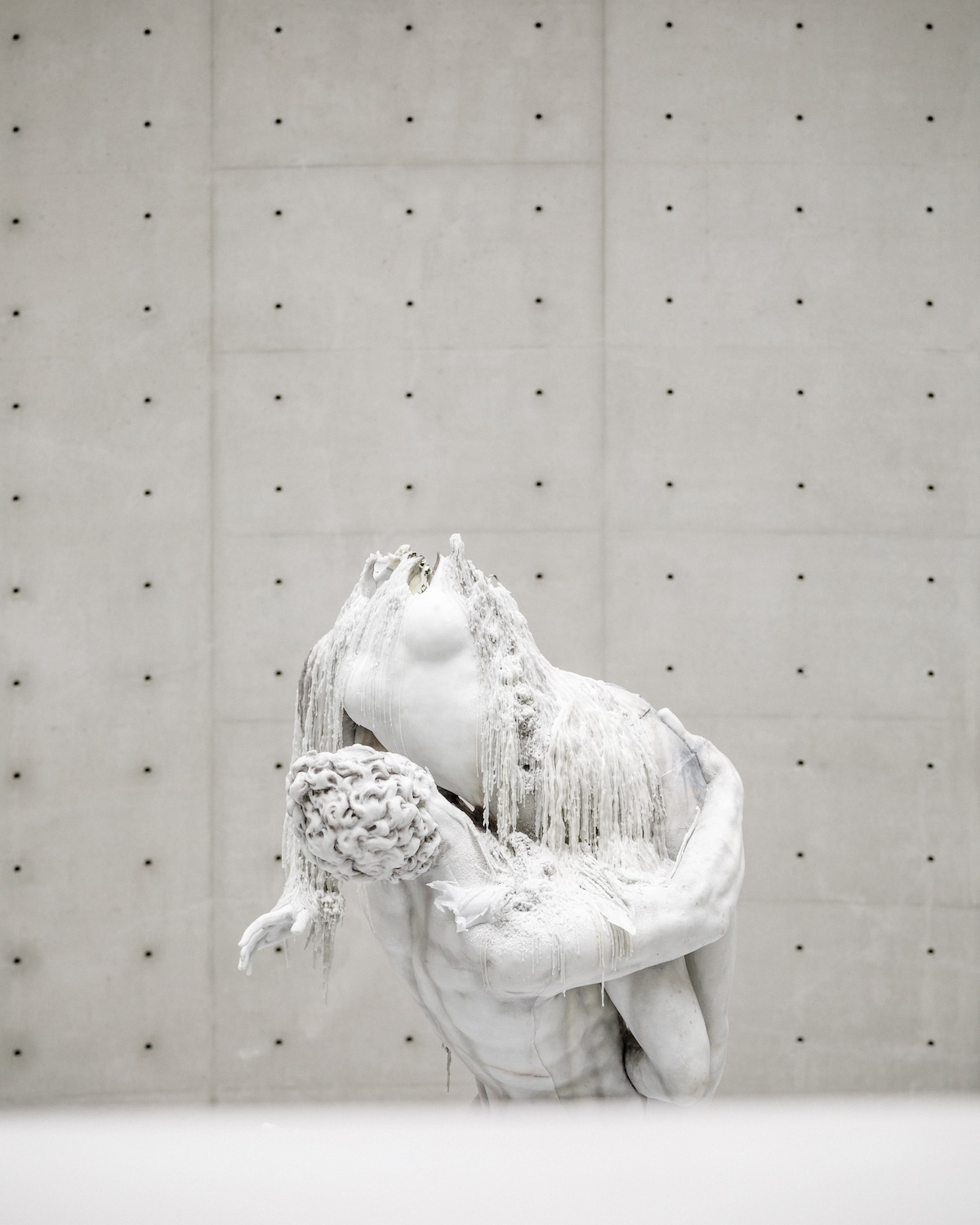In the center of the photograph stands a striking white sculpture, prominently displayed against a white tiled wall that features an array of small black holes drilled into it, resembling soundproofing patterns. This detailed marble statue depicts a muscular man, reminiscent of a figure from the Caesar era, with intricately sculpted curly hair. His back and side are visible, showing marked muscle definition highlighted in gray. The man is cradling a headless woman in his arms, her torso contorted in a position suggesting she leapt into his embrace. His left hand grips her outward-arched left hip, while her bent legs and left arm drape dramatically across him, with her right hand resting just behind his head. The sculpture exudes a fluidic, almost melted appearance, with the woman's form seeming to drip like frozen water, accentuating the surreal, ethereal quality of the artwork. The background's visual noise contrasts sharply with the intricate details of the statue, enhancing the focus on the intimate, yet fragmented, embrace between the two figures. The photo’s lower portion is blurred, perhaps due to a depth-of-field effect, drawing the viewer's attention directly to the sculpture's emotional and physical dynamism.